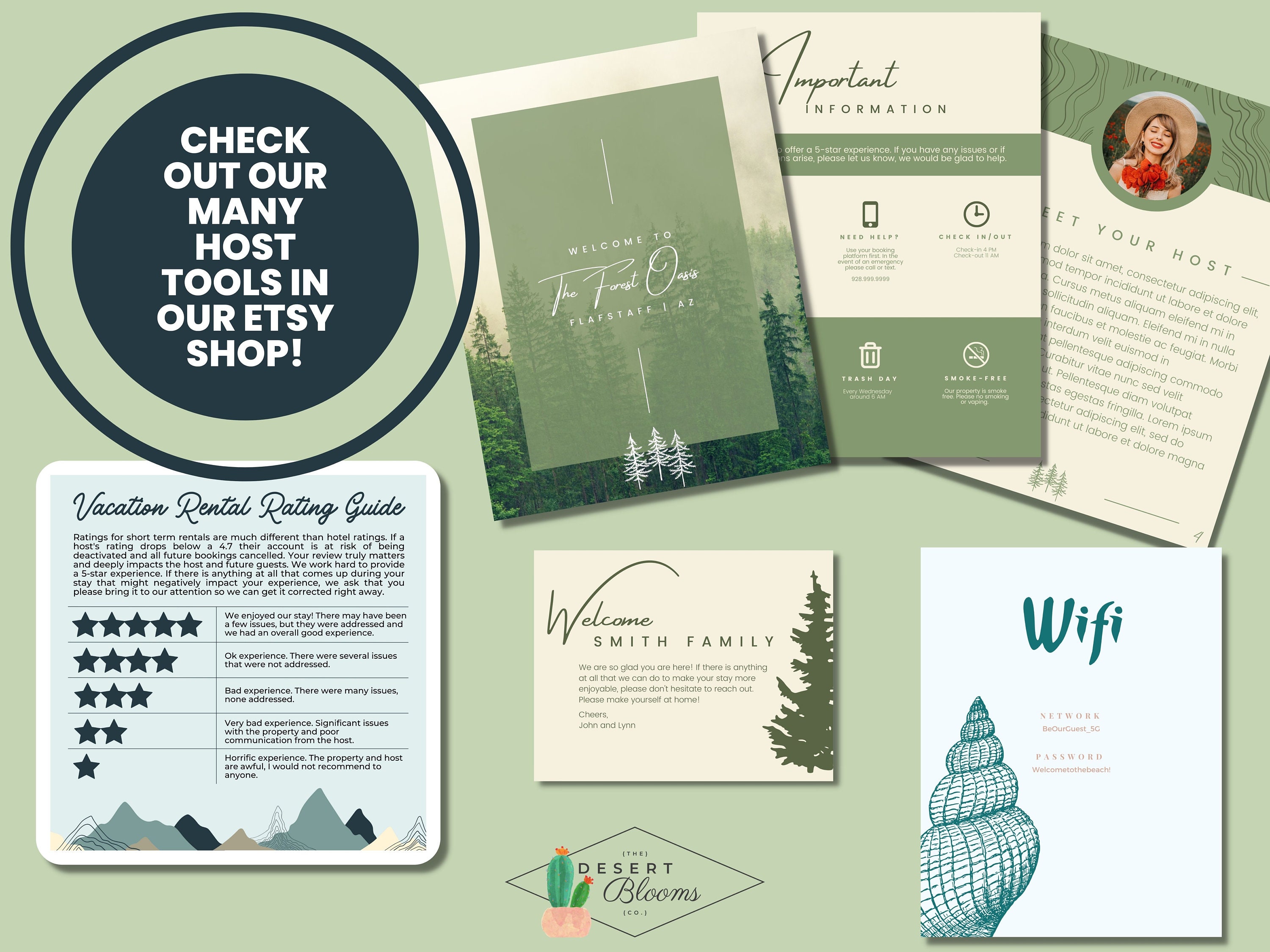In this image, set against a light green background, various colorful elements are prominently displayed, resembling cards of some sort. 

In the upper left corner, there is a large circle outlined in black, enclosing a mint-green background with a dark circle at the center. Inside this dark circle, white block text reads, "Check out our many host tools in our Etsy shop."

Positioned in the lower center of the image is a logo featuring an illustrated succulent plant in a pink pot. The succulent sits in front of a diamond-shaped background. Gray text next to the diamond reads, "Desert Blooms." 

Surrounding the logo, several greeting cards and informational cards are arranged. In the lower-left portion of the image, there is a white square with a gray interior square. The text within this square reads, "Vacation Rental Reading Guide," accompanied by an icon symbolizing a five-star rating guide below. 

The overall composition is filled with various elements, each contributing to an organized yet colorful display that highlights different aspects of what appears to be a promotional image for an online shop specializing in host tools and greeting cards.